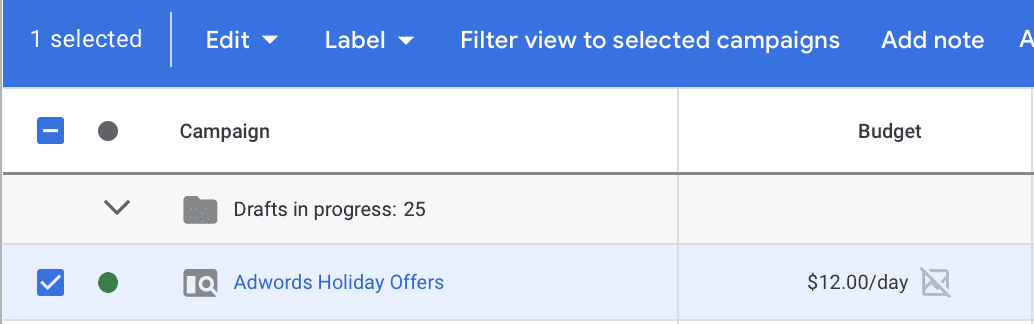Set against a solid white background, this screenshot features a top horizontal blue banner adorned with white text. From left to right, the banner displays the following elements: "Numeric 1 selected," followed by a small vertical white line. Next is "Edit" with a pull-down menu, and adjacent to it, another pull-down menu labeled "Label." Further along the banner are the options "Filter view," "To selected campaigns," and "Add note." 

Below the blue banner, on a white line, the word "Campaign" appears prominently in black text. To the left of "Campaign" is a blue box containing a minus sign. To the right, in another column, the term "Budget" is displayed. Below this section, there is a downward arrow followed by a dark gray file icon. Next to this icon, the text "Drafts in progress 25" is visible.

Finally, beneath this, a blue line features a checked white checkmark inside a blue box on the left. To its right, the text reads "Ad Words Holiday Offers." In the adjacent column to the right, the budget is noted as "$12 a day."